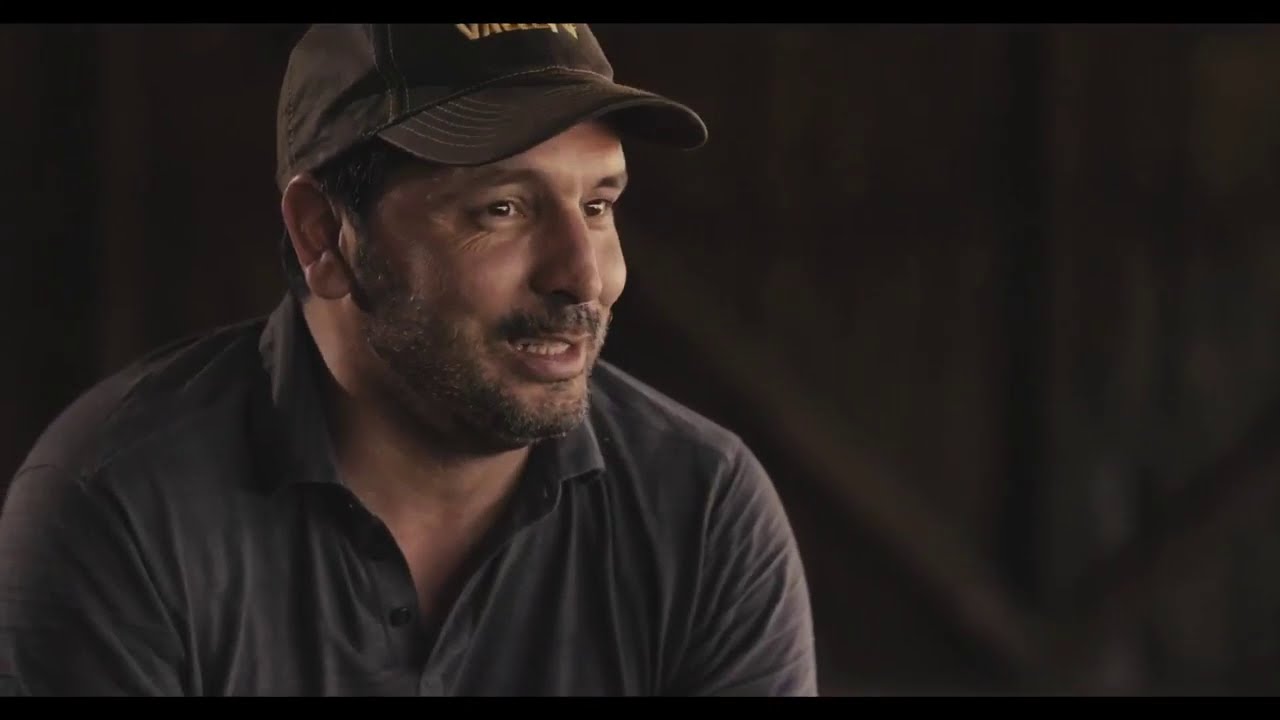In this image, we see a middle-aged man, around 40 years old, who appears to be captured in a screenshot or photograph, possibly from a video or interview. He is wearing a brown baseball cap featuring an indistinct yellow, capitalized logo and a gray collared polo shirt with some buttons unbuttoned at the neck. The man has a light brown beard and mustache, and he is smiling slightly, likely while speaking. His gaze is directed slightly to the right side. The background is blurred but seems to consist of a dark-colored sheet or wall with wooden planks forming a cross-like shape, suggesting he might be indoors in a rustic or barn-like setting. The overall composition hints at an informal, candid moment during what may be a conversation or storytelling session.